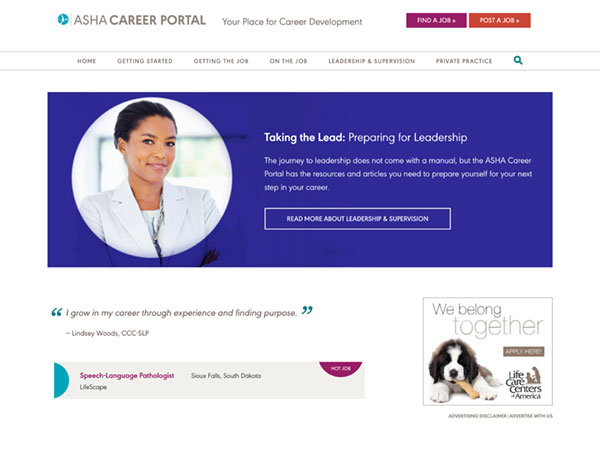Here is an improved and detailed caption for the image of the ASHA Career Portal website:

---

The image features the ASHA Career Portal homepage. In the upper left-hand corner, a small bluish icon with a white center is visible. Adjacent to this icon, separated by a vertical line, the text "ASHA Career Portal" is prominently displayed. Central to the page is the tagline "Your Place for Career Development," followed by options labeled "Find a Job" and "Post a Job." "Find a Job" is encased in a purple rectangle, while "Post a Job" is within an orange rectangle.

Beneath this section, there is a white banner with navigational links that read: Home, Getting Started, Getting the Job, On the Job, Leadership and Supervision, and Private Practice. A search icon is situated to the right of these links. Directly below this banner, a blue section features a white circular inset containing the portrait of a woman, who appears to be of Caribbean or African-American descent. She has short hair and is wearing a white suit top. 

To the right of this portrait, the text reads "Taking the Lead: Preparing for Leadership" followed by a paragraph of introductory information and a "Read More" button inside a rectangle. Below this, there is a quote attributed to her, accompanied by a banner. The bottom right-hand corner of the page showcases an image of a puppy with the text "We Belong Together" overlayed.